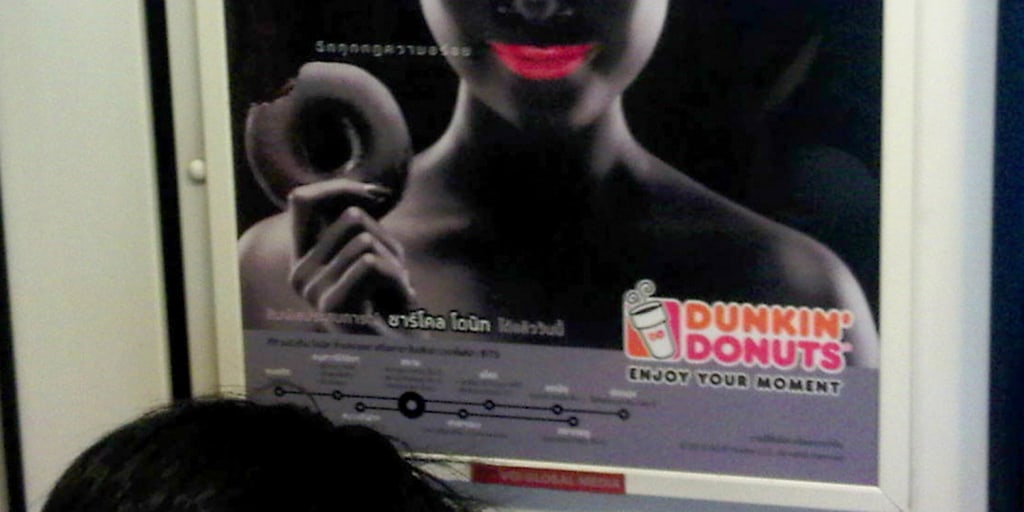In the photograph, taken indoors, there is a rectangular poster on a door, approximately six inches wide and three inches high. The poster has a thin black line running down the right-hand side and is otherwise framed by a white outline. Displaying only the lower half of a woman's face, the poster prominently features her vibrant, bright pink lipstick. She is holding a partially eaten brown donut near her face with her right hand. The text "Dunkin' Donuts" is written in the lower right corner, accompanied by the slogan "Enjoy Your Moment" beneath it, and the logo of a cup of coffee on its left.

The setting includes a door with a white wall visible on the left side, featuring a couple of vertical black stripes. Additionally, in the lower left corner of the photograph, the top of a human head with straight, dark hair partially obscures the view. The overall scene suggests a promotional environment, emphasizing the Dunkin' Donuts branding.